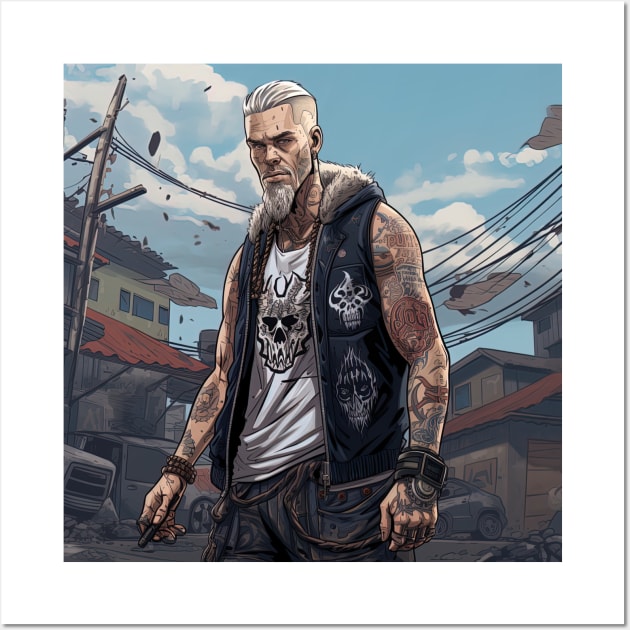The image depicts a detailed artist's illustration for a video game, showcasing a middle-aged Caucasian man with a menacing demeanor. His silver-white hair, shaved on the sides and slicked back, accompanies his distinctive facial hair—a small mustache and a long, pointed goatee. He dons a white t-shirt adorned with a skull design, layered under a black vest with a fur-lined hood also embellished with skull motifs. The man's muscular arms are covered in intricate tattoos, extending to his neck and face, emphasizing his intimidating presence. His expression is fierce, with lowered eyebrows underscoring his tough appearance. He accessorizes with a three-tiered beaded bracelet on one arm and a chunky, watch-like piece of jewelry on the other. The background sets a grim, post-apocalyptic scene: a dilapidated cityscape marred with debris, rundown cars, and houses with orange roofs under a partly cloudy blue sky. The man, striking a pose at a five o'clock angle while looking directly at the viewer, holds something cigar-shaped in his hand, asserting his prominent position in the chaotic environment.